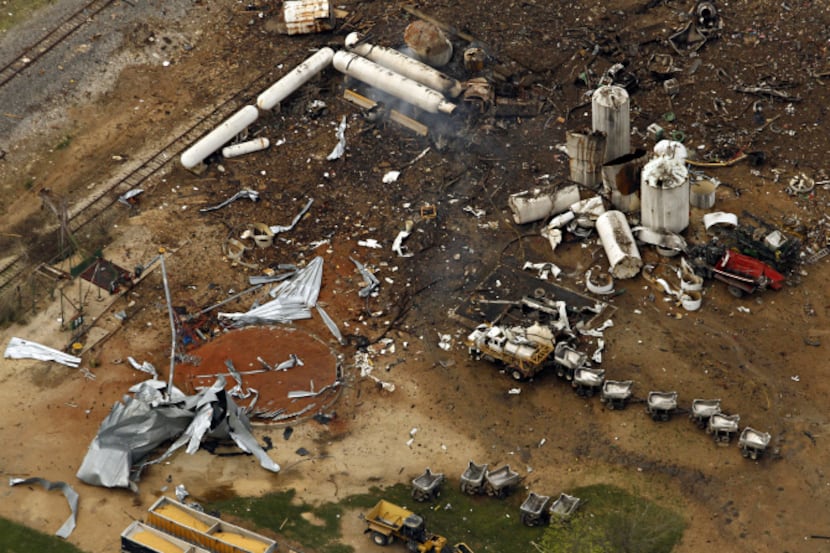This aerial color photograph captures the aftermath of a devastating explosion at a fertilizer plant. Taken from a drone in landscape orientation, the image reveals a barren, dark brown dirt area littered with debris. In the center-right, thick metal shards, possibly remnants of blown-out barrels or containers, are scattered among the wreckage. Several white barrels, some knocked over and one broken, occupy the middle-right section, while long, white, elliptical tanks, some exuding white smoke, lie on their sides towards the upper left.

A cluster of wheelbarrows, likely for cleaning, is visible at the bottom, adjacent to a line of trucks heading left. A twisted metal circular structure lies on its side, its form barely recognizable. The right center showcases several tall white cylindrical holding tanks, some bearing black char marks and fragments strewn around.

Two yellow construction trucks are hauling debris: one is in the center-right, with numerous containers of debris trailing behind it toward the bottom right, and the other is at the bottom center, surrounded by empty containers. Railroad tracks appear on the left-hand side, amidst turned-over trucks. The entire scene embodies chaos and destruction, starkly represented through photographic realism.